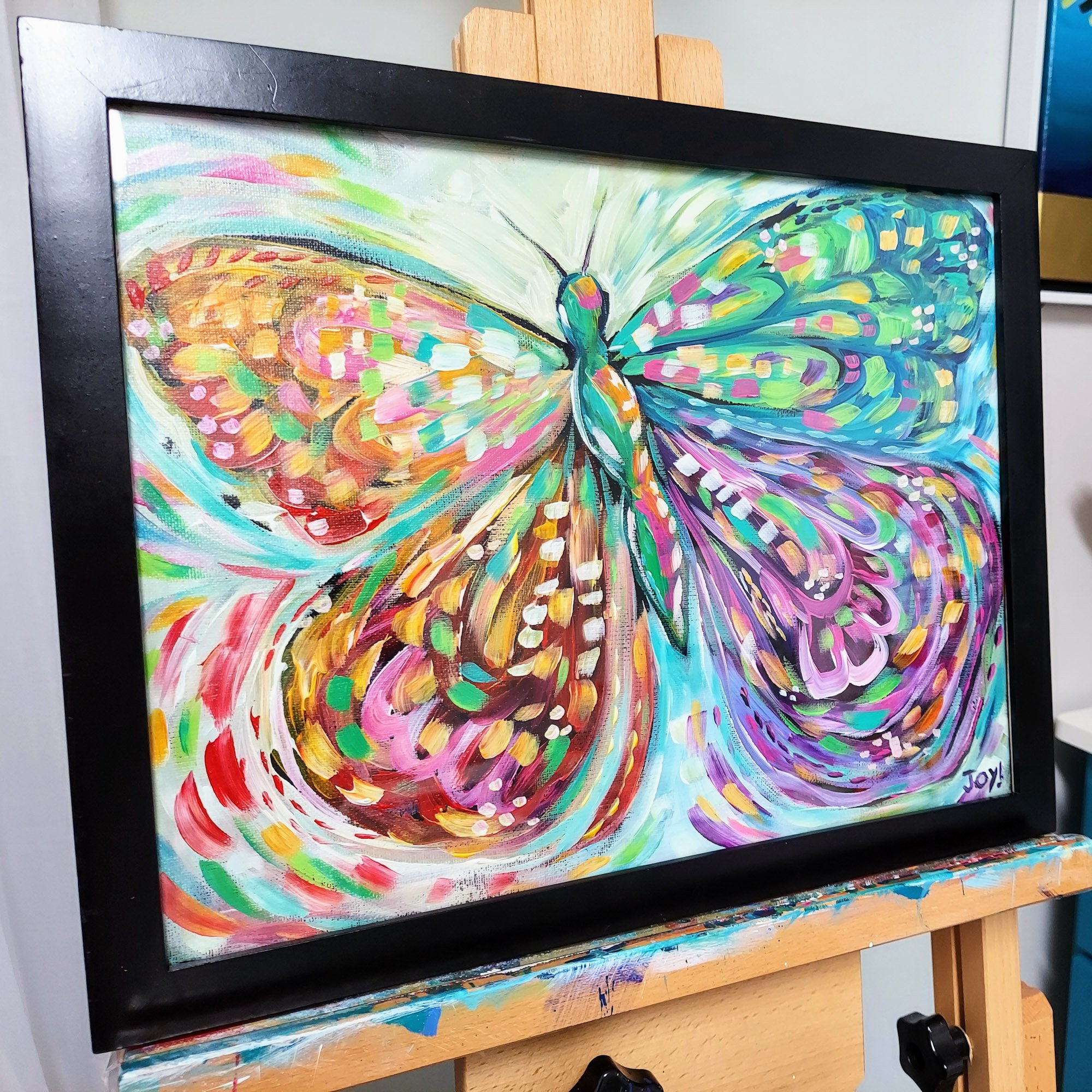The image captures a beautifully detailed framed painting of a colorful butterfly, prominently displayed on a wooden easel that's spotted with paint stains reflecting the hues from the artwork. The butterfly, painted with intricate patterns and vibrant shades of green, blue, purple, pink, white, yellow, and orange, has an eye-catching green body adorned with a yellow and pink stripe. Its wings, though asymmetrical in color, are symmetrical in shape, with a distinct pair at the front and another at the back. The butterfly’s head features two upward-extending antennae. Surrounding the butterfly is a swirling background that incorporates the same vivid colors, enhancing the composition. The painting is held within a sleek black frame, and at the bottom right-hand corner, the artist’s signature "Joy!" is visible. The easel, positioned slightly leaning and equipped with visible adjustment knobs, adds to the artistic ambiance of the scene, with a glimpse of an art studio setting in the background.